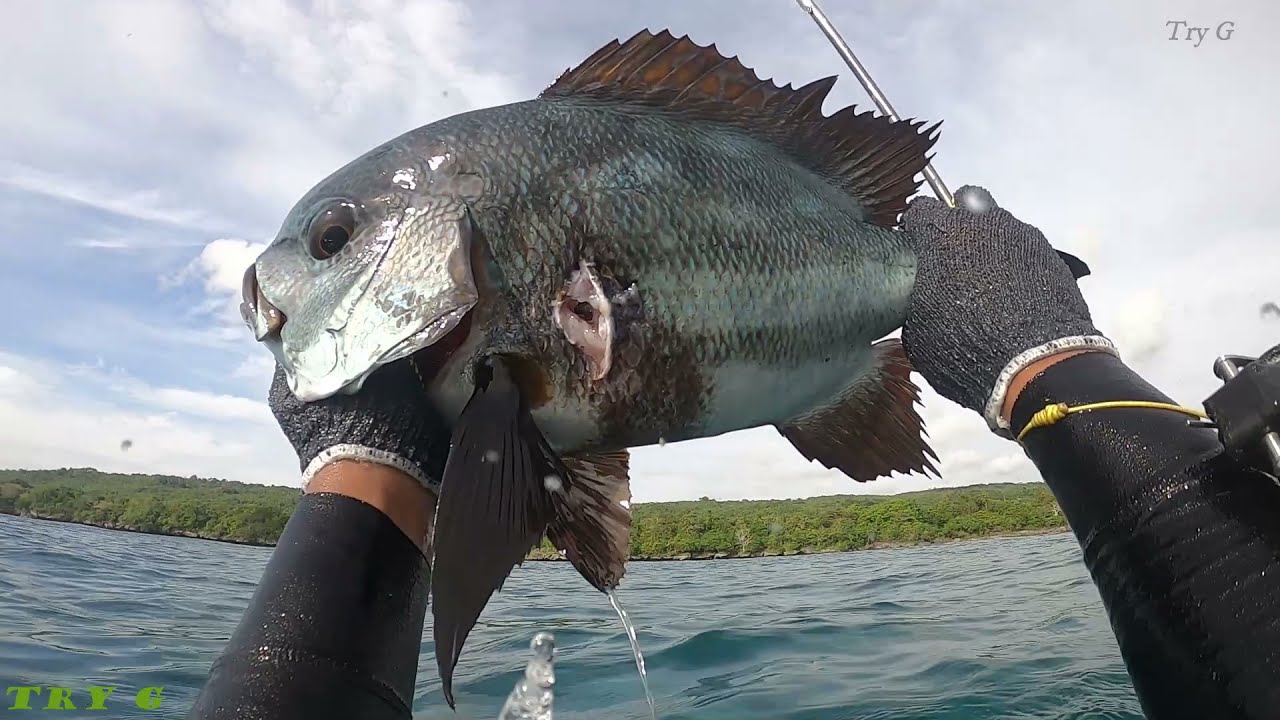In this professionally taken first-person point of view image, two hands clad in black gloves and a matching wetsuit hold up an enormous fish dripping water. The fish is predominantly gray and silver with distinctive brown accents and large, expressive eyes. The scene is set against a backdrop of a choppy blue body of water and a lush mountainous terrain covered in vibrant green trees. Above, the sky is a serene blue scattered with wispy white clouds. The fish appears stout and robust, with visible gray streaks on its back and brown fins. There is a notable chunk missing from the middle of the fish revealing its flesh, suggesting it may have been caught during a spearfishing expedition. In the upper right corner, the text "TRY-G" is visible in green.